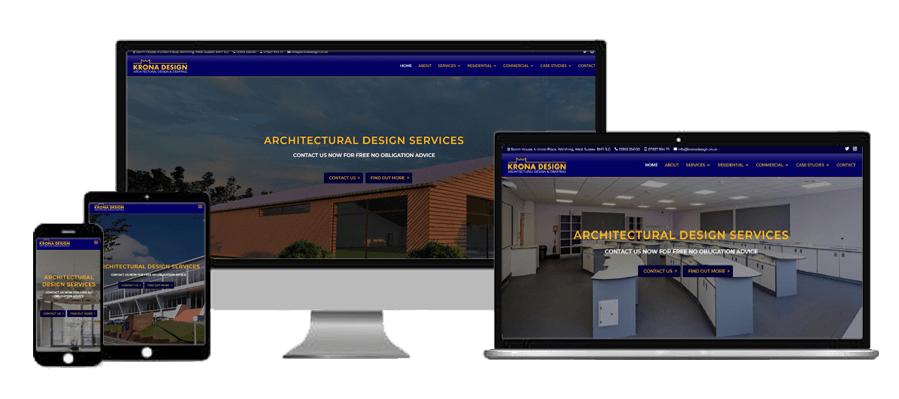This image showcases the versatility of Architectural Design Services' website across multiple devices, highlighting its adaptability and user-friendly interface. 

From left to right, the display features:

1. **Monitor:** Showing the website on a full-sized monitor, the largest of all devices displayed. The monitor screen highlights a detailed image of a building, prominently featuring the Architectural Design Services logo in vibrant yellow. Two blue navigation options are visible, emphasizing the firm's branding and user navigation approach.

2. **Laptop:** Here, the website is depicted on a laptop screen. The same Architectural Design Services logo is present, maintaining brand consistency. The featured image on this device captures an interior view of a classroom-style laboratory. The room is furnished with three rows of tables and lined with cabinets at the back, suggesting a well-organized and functional space.

3. **iPad:** The iPad display shows a different image, this time of a building that appears to be a school. The school building has numerous windows and is surrounded by neatly maintained shrubbery, showcasing the architectural firm’s ability to incorporate natural elements into their designs. The yellow logo of Architectural Design Services remains consistent, reinforcing brand identity.

4. **Phone:** The smallest screen, a cellphone, also features the same yellow logo of Architectural Design Services. Due to the limited size of the display, the image content is less discernible but serves to illustrate the mobile-friendliness and responsive design of their website.

Overall, this image exemplifies Architectural Design Services’ expertise in creating a cohesive and visually appealing online presence across various digital platforms.